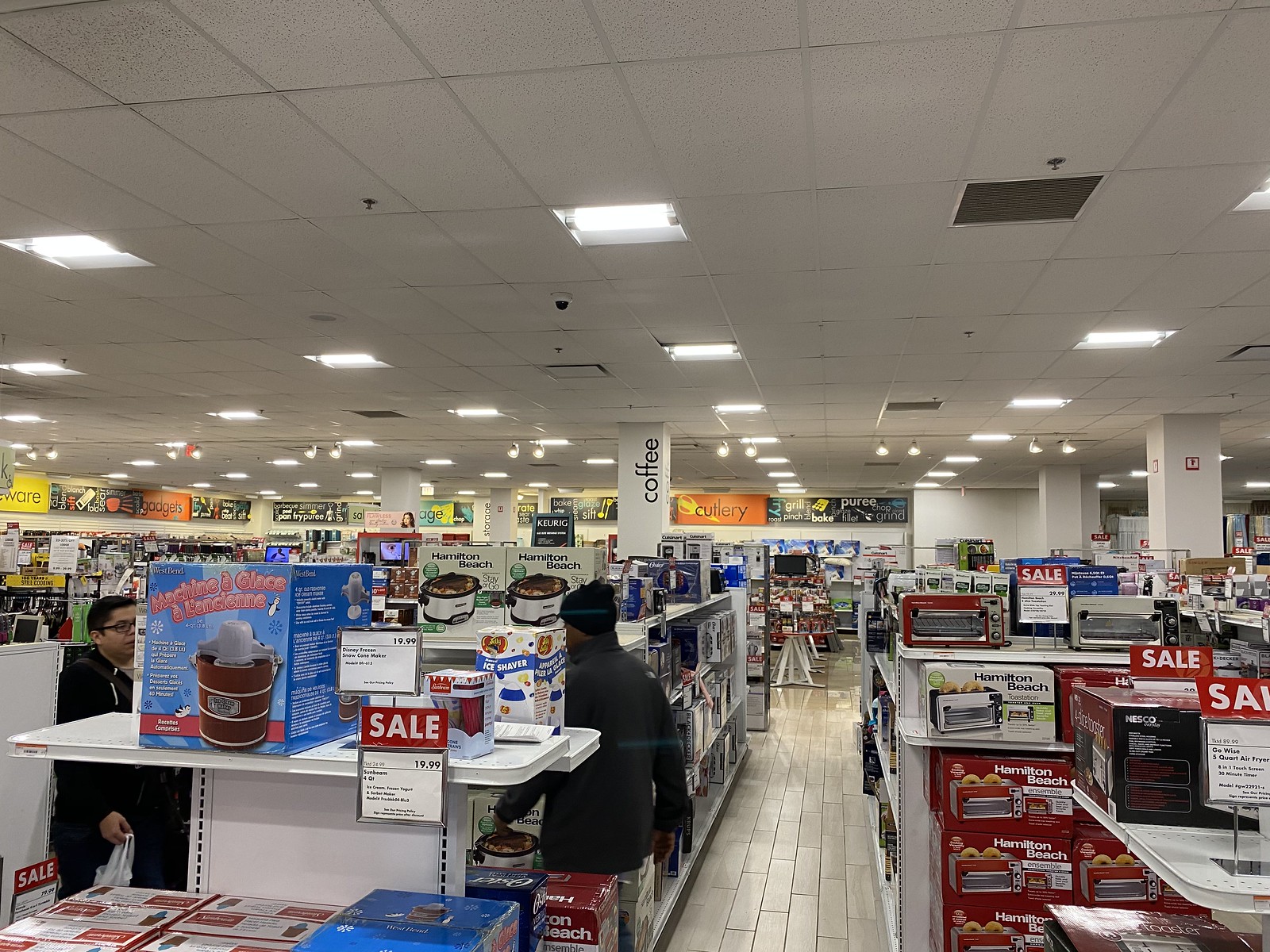Inside a vast and bustling department store, the scene is alive with activity and an array of products on display. The overhead view reveals a roof adorned with large rectangles and square lights that shine brightly, casting a white light over the sprawling aisles below. The roof itself has a rough, crunchy texture. Dominating the lower half of the image are white shelves brimming with merchandise. Prominently featured are Hamilton Beach appliances, including toaster ovens and a central crock pot.

To the left side of the composition stands an ice cream machine in a blue box, which captures the attention of a man wearing glasses. Nearby, another man stands with his back to the camera, both of them engrossed in the items. Scattered throughout the store are numerous red sale signs emblazoned with the word "Sale" in white, adding to the bustling atmosphere.

In the distance, distinct signage helps guide shoppers: a large white pillar marked with the word "Coffee" in black writing, and two rectangular posters—one with an orange background reading "Cutlery" and the other with a black background spelling out "Puree." The image conveys the vastness and consumer variety of the store, filled with countless products and vibrant sale promotions.